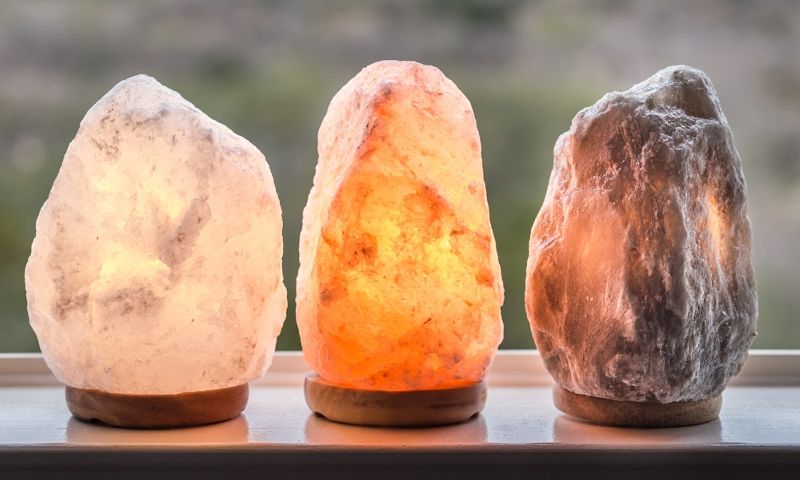The image depicts three luminescent crystals, likely Himalayan salt lamps, elegantly showcased on a white, possibly marble windowsill. Each lamp features a distinct coloration and rests on a simple, flat, circular wooden stand. The lamp on the left is predominantly white with subtle gray streaks, exuding a soft, translucent glow that resembles lit marble. The center lamp radiates a warm orange hue, indicating it's illuminated from within. The lamp on the right is a deep, nearly opaque dark gray, with only faint hints of light piercing its surface. The blurred background hints at greenery or trees, enhancing the focus on the three vibrant lamps.